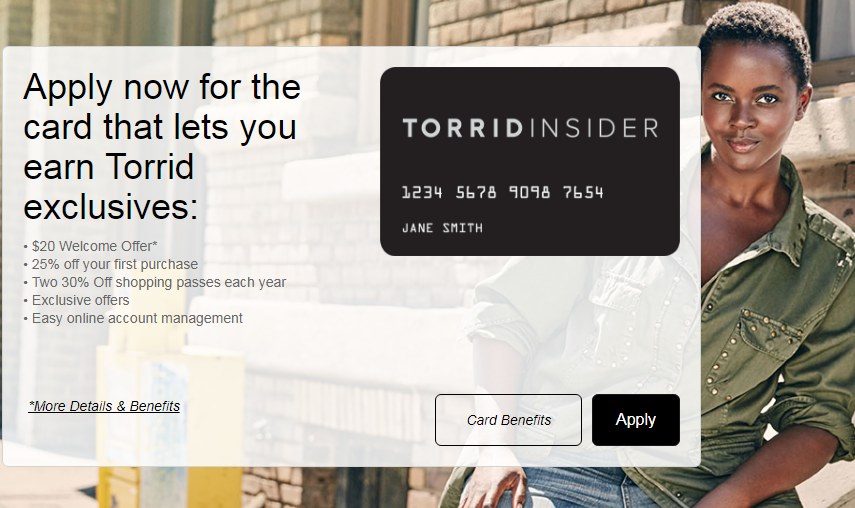In the background of this image, there's a large brick building stretching across the entire scene. On the right side of the image, there's an African American woman with very short hair, smiling softly without showing her teeth. She is wearing a green shirt and blue jeans. Part of her body is obscured by a box in the foreground. Behind her, a noticeable yellow object adds a splash of color to the scene.

Overlaid on the image is a semi-transparent white rectangle, allowing the building, the yellow object, and part of the woman to remain visible. The rectangle contains black text promoting a card. It reads: "Apply now for the card that lets you earn Torrid exclusives." Below this headline are five bullet points detailing the card's benefits:
1. $20 welcome offer
2. 25% off your first purchase
3. Two 30% off shopping passes each year
4. Exclusive offers
5. Easy online account management

At the bottom of this overlay, beside a star indicating more details about the welcome offer, it states "More details and benefits," which can be clicked. Beneath this, an image of a card labeled "Torrid Insider" is displayed, with "Card benefits" written below it. At the very bottom, there's a black button that reads "Apply."